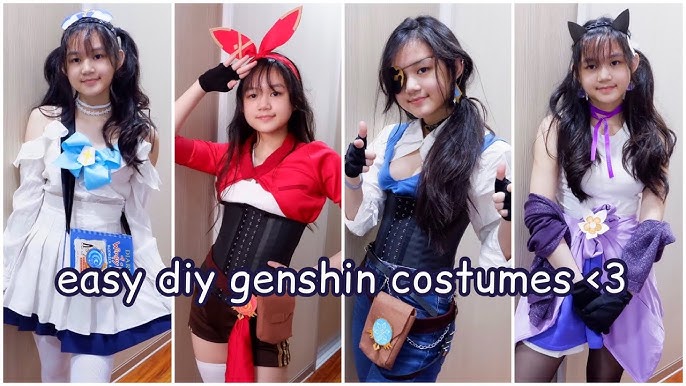This image is a rectangular photo collage featuring the same person in four different DIY Genshin Impact costumes. The overlay text reads "Easy DIY Genshin Costumes" followed by a heart symbol created using the "less than" sign and the number three (<3). The first photo shows her in a blue and white dress with long sleeves, complemented by black gloves and a headpiece. In the second photo, she's wearing a red bolero top over a black corset, with white stockings and red bunny ears. The third costume features a pirate-inspired look: a blue and white dress with black accents, an eye patch, fingerless gloves, and a brown pouch. Finally, the fourth outfit consists of a white top, a light purple and purplish-blue skirt, black tights, lavender scarf, and black cat ears with her hair styled in two ponytails. The model appears to be of Eastern Asian descent.